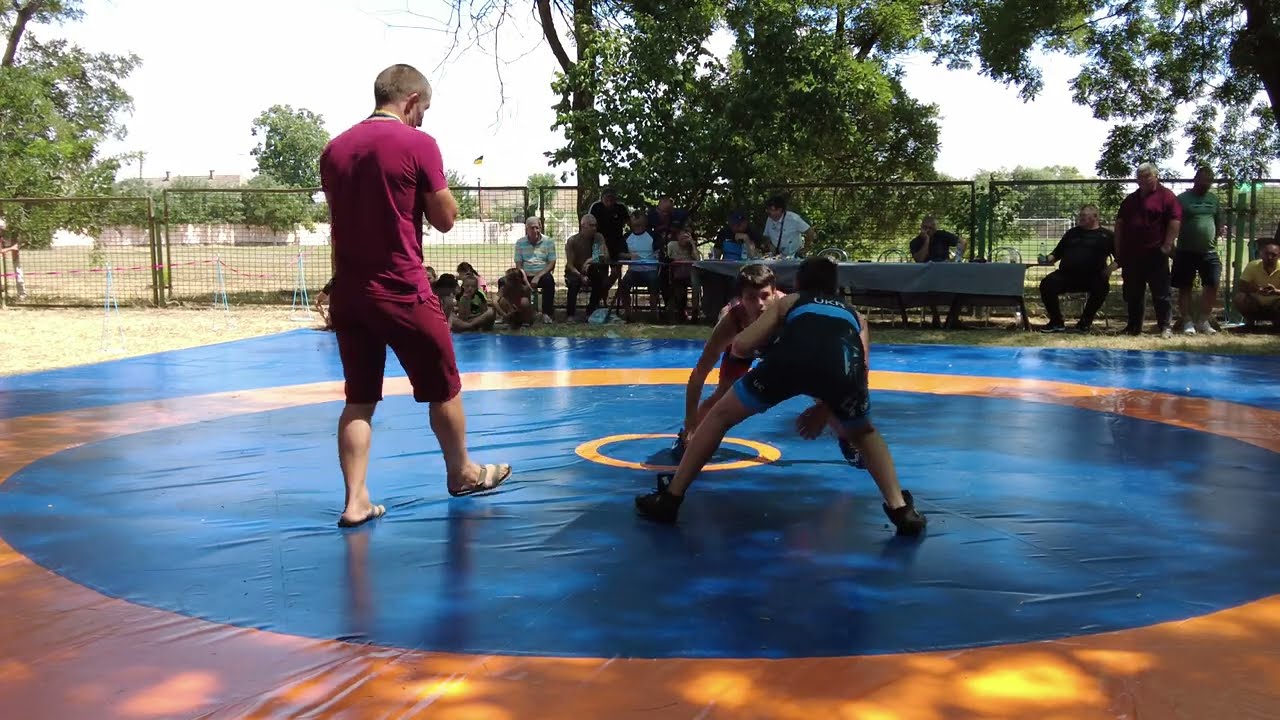This outdoor daytime photograph captures what appears to be a high school wrestling match set in a backyard or enclosed park area. Dominating the scene is a large collegiate wrestling mat featuring a central blue circle surrounded by wide yellow rings and blue outer edges. Positioned at the center of the mat, two Caucasian teenage wrestlers are engaged in a match. The one facing away from the camera wears a dark blue and light blue singlet, his legs spread wide in a crouched, ready stance. Opposite him, another boy mirrors this stance, identifiable by his red jersey. 

Overseeing the match is a referee, distinguished by his maroon short-sleeve shirt and shorts, standing on the left side of the wrestlers. He wears white shoes and has his back to the camera. Surrounding the wrestling area, a group of spectators of all ages are seated on the ground, in chairs, and behind a long table against a chain link fence that spans the background from left to right. The fence demarcates this wrestling area from a larger field dotted with various trees beyond. The atmosphere suggests a casual, community event, possibly involving picnicking or barbecuing, given the mixed setup and gathering of people.